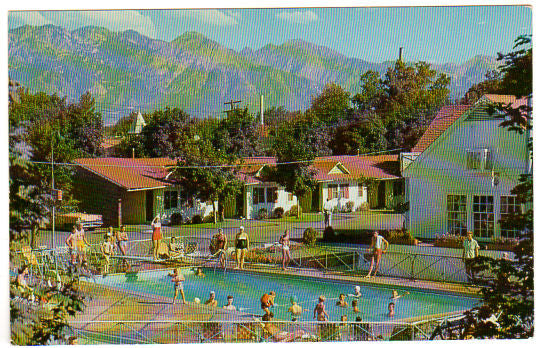The image depicts a grainy, possibly vintage photograph or drawing of a busy community pool from what appears to be the 70s or 80s. The long rectangular swimming pool is situated within a fenced area. Surrounding the pool are numerous adults and children, many wearing colorful bathing suits, either swimming or standing around. The background features rows of small, white houses with red or orange roofs, and a larger, two-story white building with French doors that might be a community center. Behind these homes are tree lines and a mountain range under a blue sky with some clouds. The overall image has a yellowish tinge and a pixelated, grainy quality, possibly due to age or water damage, giving it a nostalgic feel.